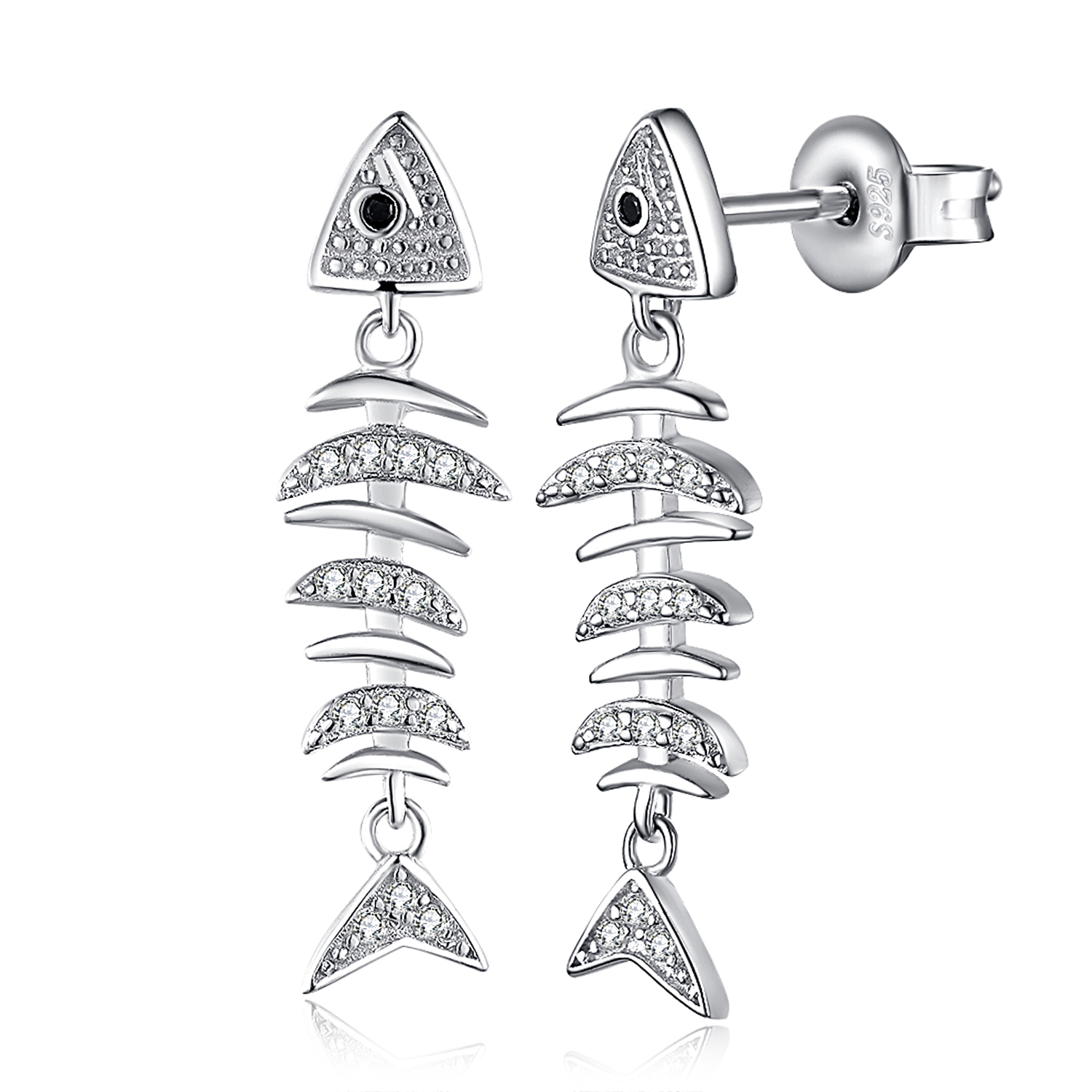The image depicts a high-quality commercial photograph of two intricately designed fish-shaped earrings, crafted from silver metal. Both earrings are displayed in a clear, edge-to-edge view. The fish design begins with a triangular fish head, adorned with a small black gemstone as the eye, and continues down the body with alternating segments of bare metal and diamond-encrusted sections in a pattern reminiscent of fish scales and bones. The lower sections of the fish's body include small half-circle pieces, ending with a detailed tail. On one earring, the post and earring back are visible, inscribed with "S925", indicating sterling silver. The meticulous detailing and sparkling rhinestones suggest that this image could likely be used for an advertisement or catalog to showcase these elegant pieces of jewelry.